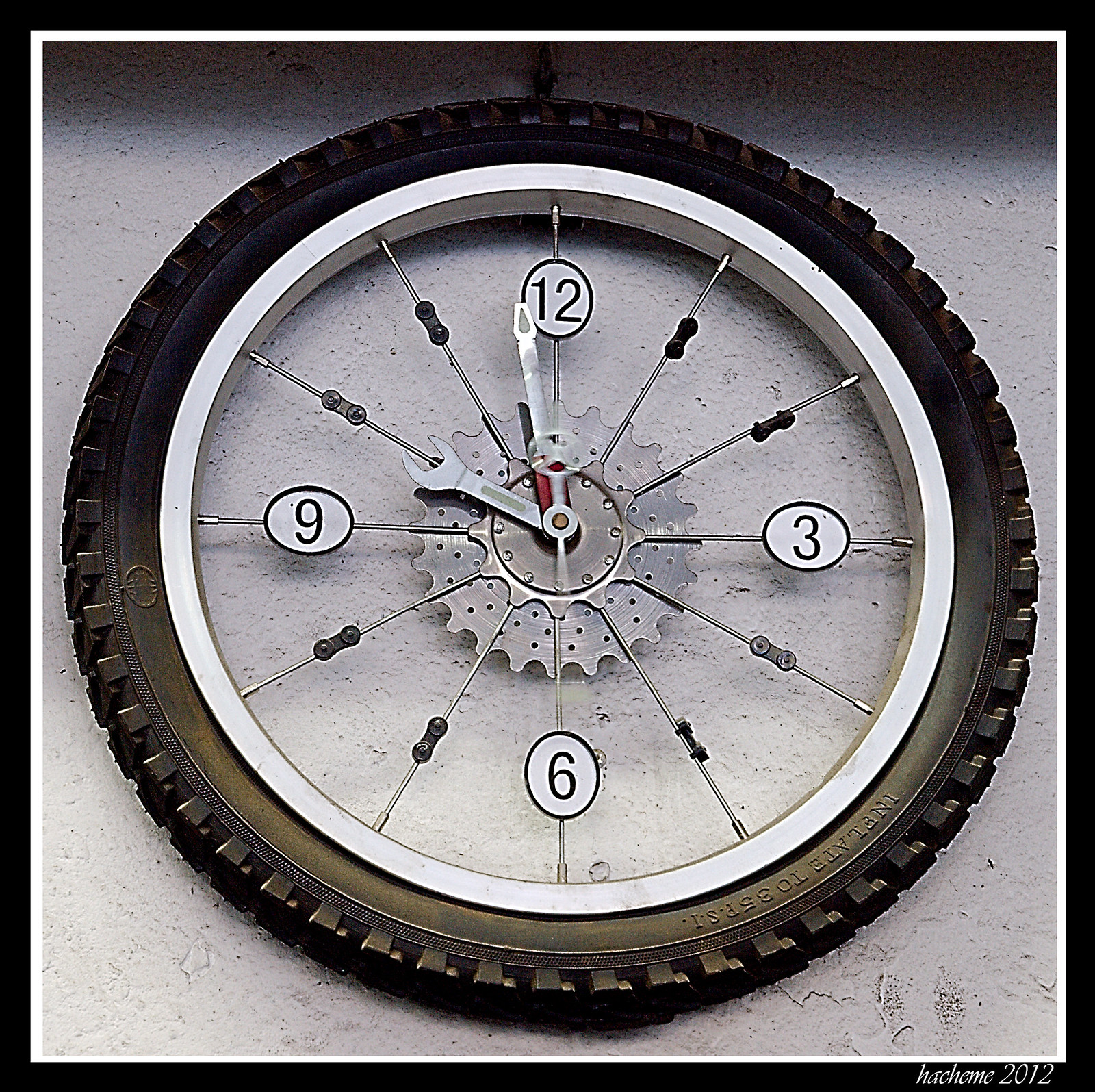The image shows a close-up of a highly unusual wall clock designed to resemble the inside of a tire. The clock face is encased within a black tire-like frame that features tread and a white rim. The clock face, which is mostly light gray with splotches that give it a weathered look, is designed to mimic the wheel of a bicycle, with spokes radiating from the center. Only the numbers 12, 3, 6, and 9 are displayed on the clock face, each positioned on metallic, silvery background elements. The hour and minute hands are crafted in the shape of tools; one is a spanner, and the other is a screwdriver. The clock appears mounted on a silvery wall with peeling paint, and the entire scene is framed in black. At the bottom of the image, there is a name followed by the year 2012, adding a final touch to the unique piece.